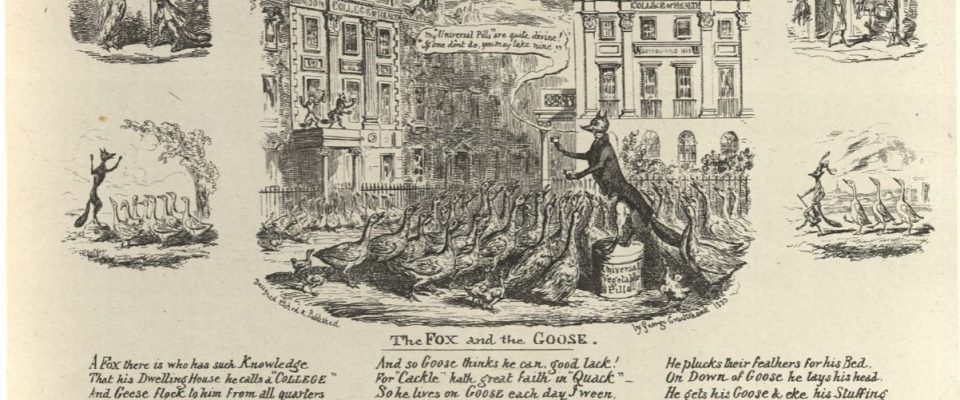A detailed black and white vintage illustration, potentially dating from the mid-1800s to early 1900s, resembling a classical book illustration or old comic strip. The central image depicts a fox, dressed in a suit or tuxedo, standing on a pedestal and giving a speech to a gathering of attentive geese in front of a grand classical architecture building that resembles a government structure. Beneath the main image, the title "The Fox and the Goose" is inscribed along with a passage of elaborate, antiquated English text. It reads, "A fox there has such knowledge that his dwelling house he calls a college and geese flock to him from all quarters and so goose think he can he can good luck for cackle hath great faith in quack so he lives on goose each day when he plucks the feathers from his bedder on down of goose he lays his head he gets his goose his stuffing." Surrounding the main image are smaller vignettes: one side image shows the fox, staff in hand, leading the geese away, while another depicts the fox delivering a speech to the geese in an outdoor setting. The series conveys a narrative of the cunning fox deceiving the geese to follow him, symbolizing manipulation and deception.